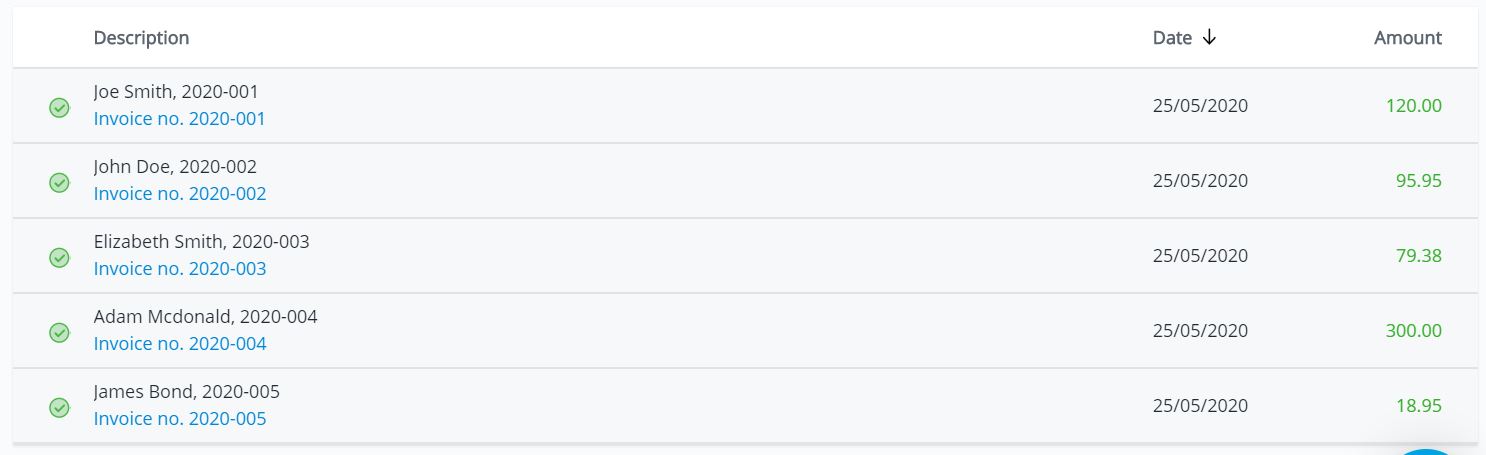In the image, we observe a detailed section of an invoice page, likely from a phone application. The layout is systematic with headers and entries prominently detailed. At the top, there is a header row with columns labeled "Description," "Date," and "Amount." Below this, five entries with accompanying details are meticulously listed.

1. **Joe Smith**: Invoice number 2020-001, dated 25-05-2020, with an amount of $120.00.
2. **John Doe**: Invoice number 2020-002, dated 25-05-2020, with an amount of $95.95.
3. **Elizabeth Smith**: Invoice number 2020-003, dated 25-05-2020, with an amount of $79.38.
4. **Adam McDonald**: Invoice number 2020-004, dated 25-05-2020, with an amount of $300.00.
5. **James Bond**: Invoice number 2020-005, dated 25-05-2020, with an amount of $18.95.

The amount figures are highlighted in green, adding emphasis to this specific column. Each description entry has a green check mark adjacent to it, suggesting completed transactions or verified entries. The overall design employs a clean, gray-and-white color scheme, ensuring the highlighted elements stand out for quick reference.